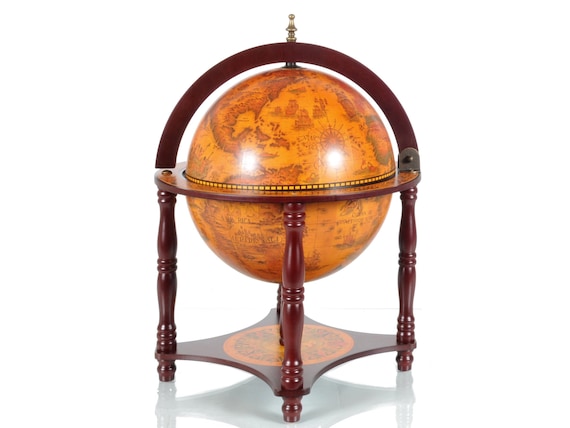The image showcases an antique-looking globe set against a completely white background. The globe, rendered in muted shades of red, orange, and brown, outlines various countries without any visible lettering. It rests on an elegant wooden stand, likely mahogany or cherry red in color, composed of four curvy legs attached to a small base. This base is primarily wood-toned with an orange circle at its center. The stand features a wooden strip that arches over the top of the globe, culminating in a small gold spindle. The overall design suggests the globe is capable of spinning. A subtle shadow or reflection is visible beneath the stand, adding depth to the scene.